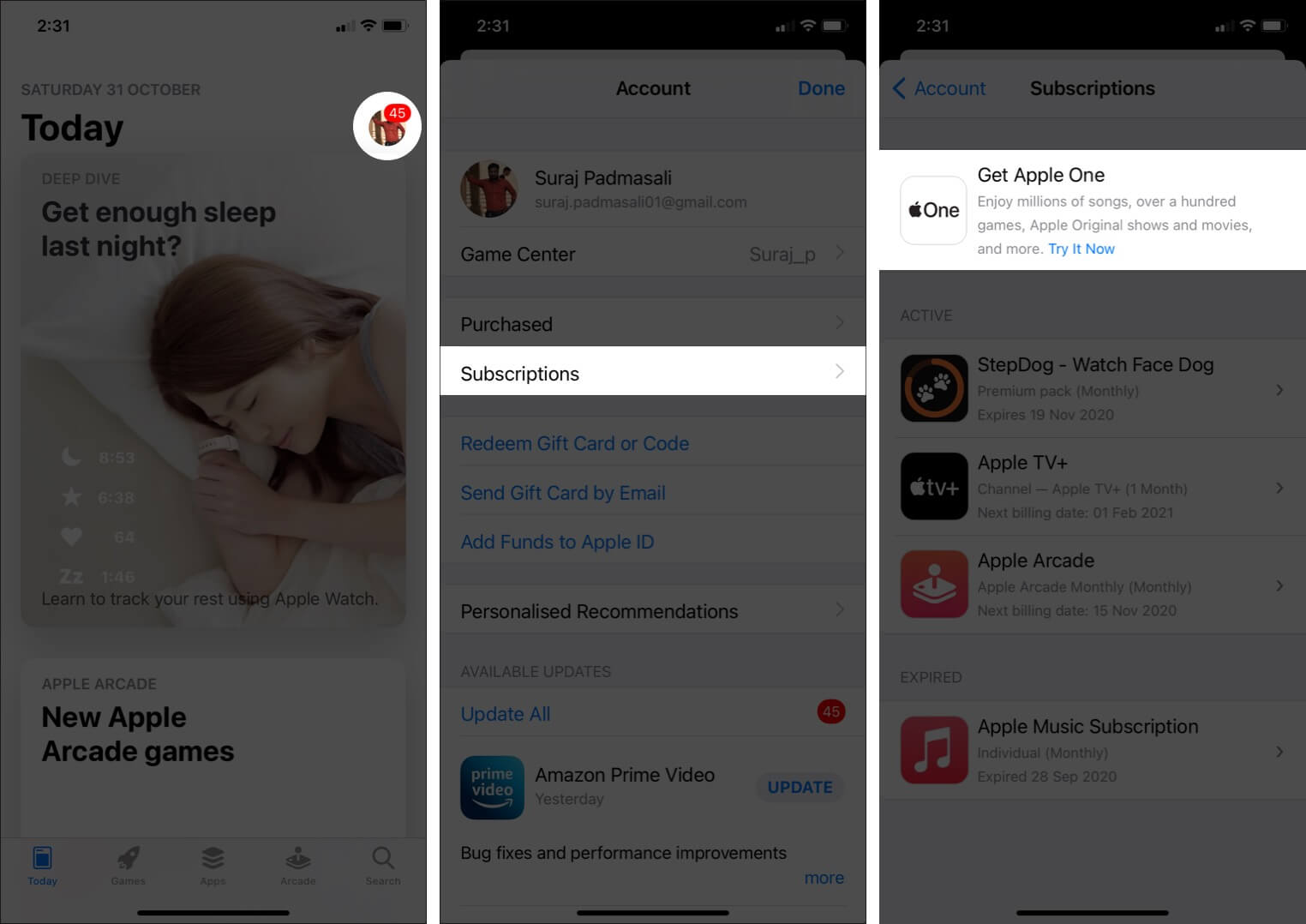The image displays three screenshots of a smartphone interface, presumably taken from a website about sleep. All three screenshots have a gray overlay, indicating they are not active or selected, except for certain highlighted areas which are white. The details of each screenshot are as follows:

1. The first screenshot shows a webpage under the title "Today," dated Saturday, October 31st, at 2:31. The page features various segments including "Deep Dive," "Get Enough Sleep Last Night," and "New Apple Arcade Games." The top of the screen displays standard mobile indicators such as cell reception bars, battery level, and data connectivity.

2. The second screenshot has the account page of a user named Suraj Padmasali. The Game Center interface is displayed with a focus on the "Subscriptions" section, which is highlighted in white while the rest of the page is faded in gray.

3. The third screenshot again focuses on the "Subscriptions" section, specifically highlighting an option to "Get Apple One," which offers a bundle including millions of songs, hundreds of games, Apple original shows and movies, and more. This selection is white and prominently displayed against the gray background of the page.

Together, these screenshots seem to emphasize details about account management and subscription options, particularly highlighting Apple's services.